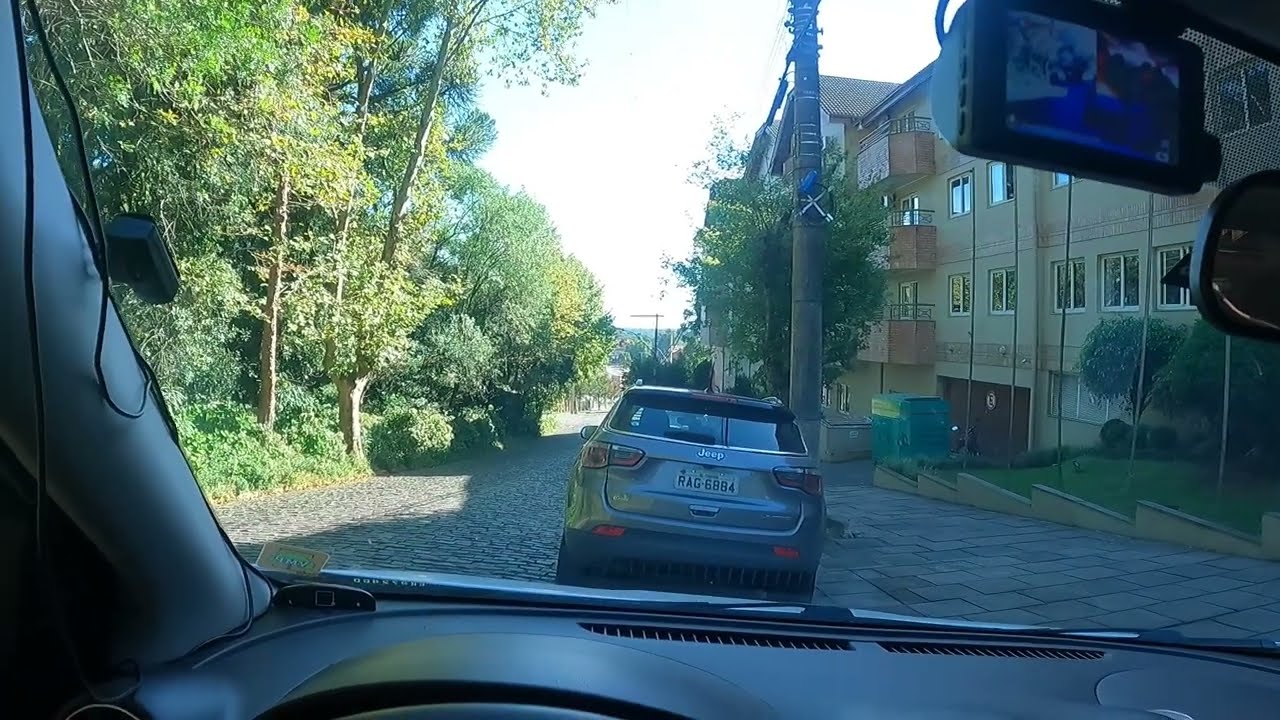The image portrays a detailed view from inside a stationary vehicle, likely taken from the front left-hand seat, either driver's side if the driver sits on the left, or passenger's side if not. The vehicle's black dashboard and a portion of the windshield are visible, along with the left edge of the rearview mirror and a heads-up camera display situated above and to the left of it. The scene outside reveals a cobblestone street bordered by a stone sidewalk. Directly ahead, there is a gray hatchback vehicle which seems stationary as well.

To the left of the cobblestone street extends a grove of tall, green deciduous trees, indicating a spring or summer setting. The dense wooded area stretches off into the distance. On the right side of the street, a cream-colored building with at least three stories rises. This structure, possibly an apartment building or hotel, features balconies with brown railings on its upper floors, specifically the second, third, and fourth levels. The bright sky enhances the overall brightness and clarity of the scene, reinforcing a clear, sunlit day.